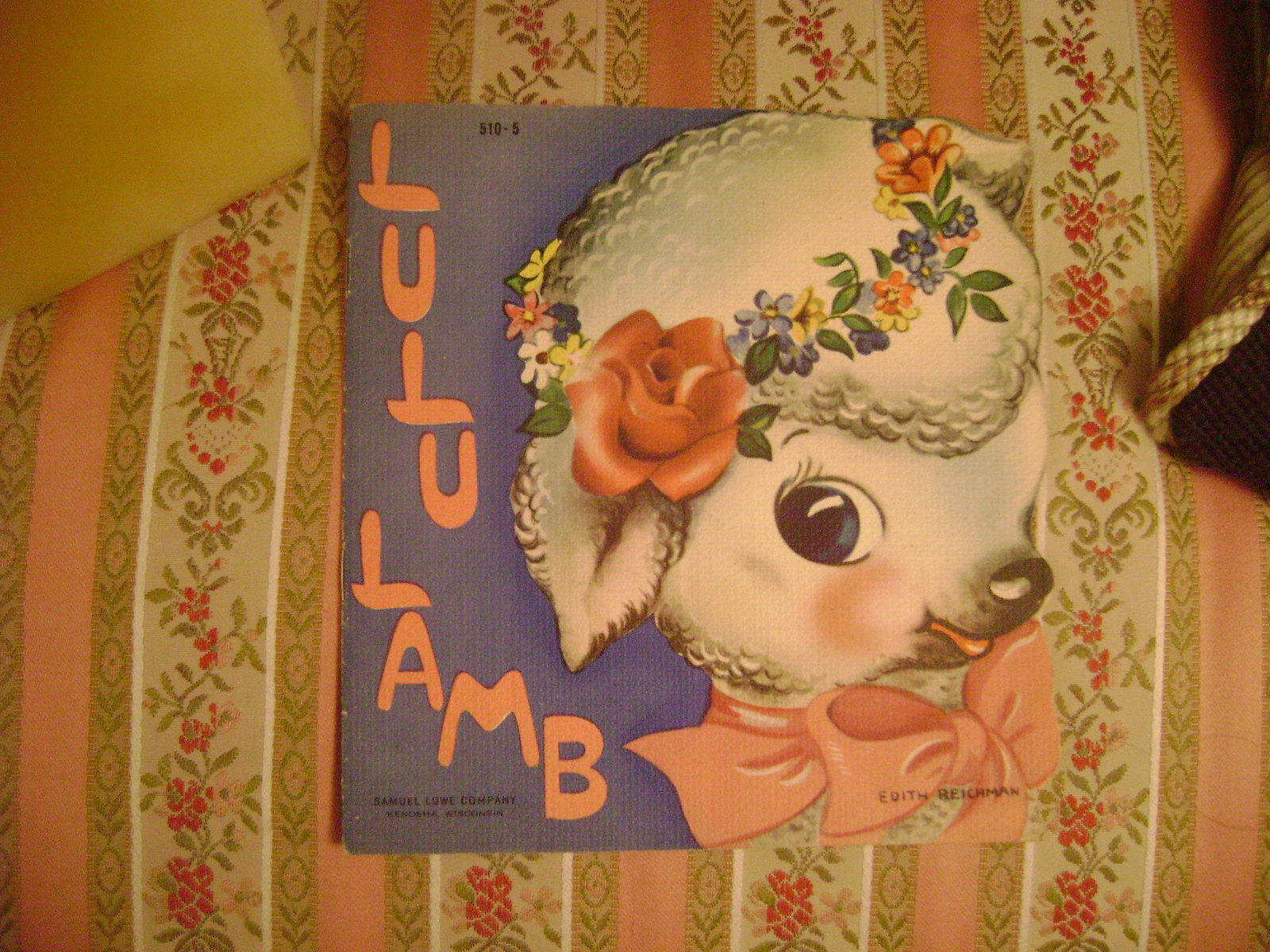The image depicts a photograph of a square book or paper titled "Lulu Lamb," featuring an illustration of a white lamb with black markings near its face. The lamb's head is adorned with colorful flowers, including a prominent rose, and a red bow around its neck. The lamb has one visible blue eye and an open mouth, giving it a friendly appearance. Additional text, "Samuel Yoke Company" and "5105," is seen on the document, with a blue background.

This object is resting on a couch with a distinctive, dated vertical stripe pattern. The pattern alternates between pink stripes, gold stripes with green leaves, and another tan stripe with additional flowers and leaves, repeating this sequence across the fabric. The full pattern appears four times in the visible section of the couch. The photograph also reveals part of a yellow pillow in the top left corner and a partial view of a brown and white object on the right side. The floral motifs on the couch and the lamb's head seem to blend together, enhancing the overall aesthetic coherence of the image.